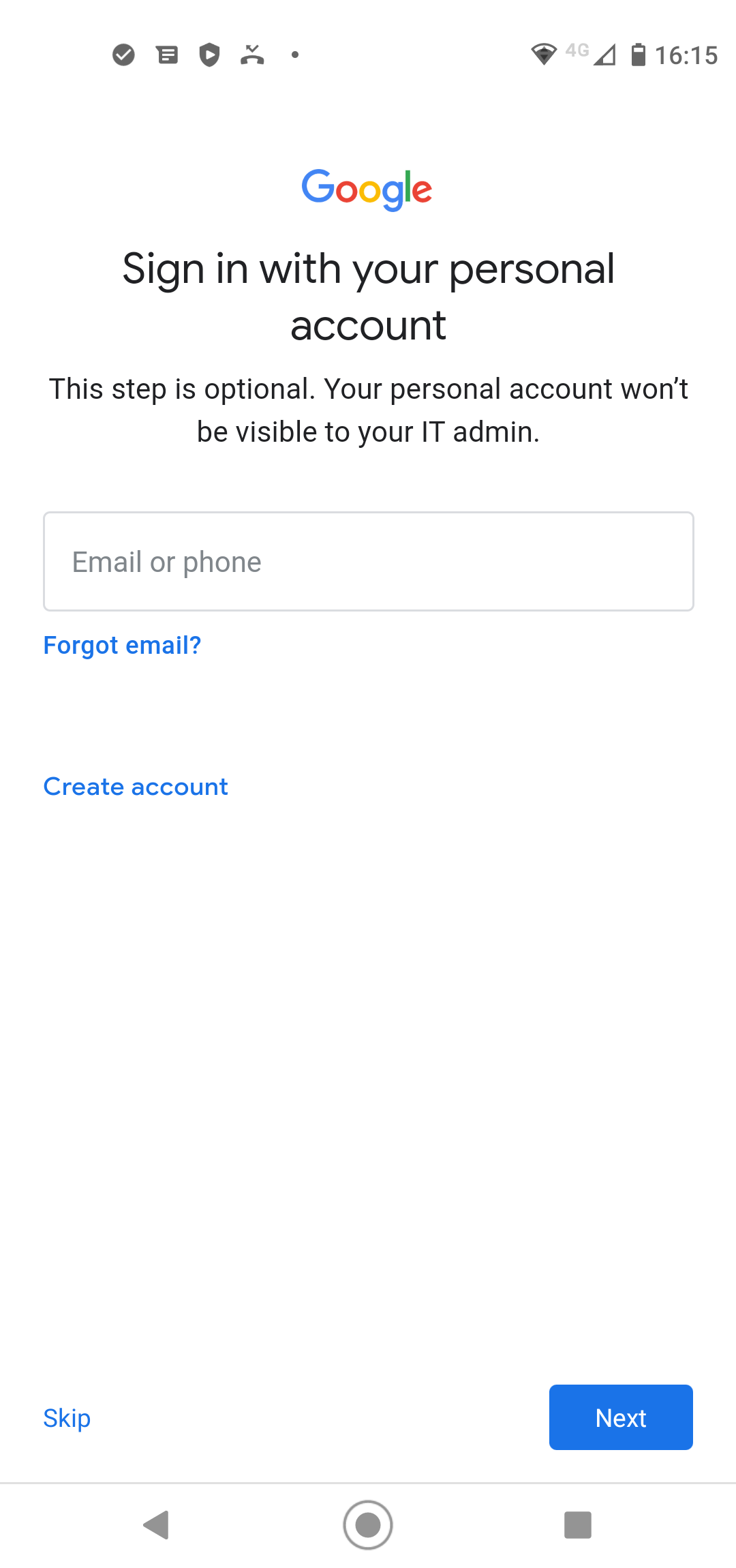A detailed vertical screenshot of an individual's smartphone displaying the Google sign-in page. At the top, the distinct Google logo with blue, red, yellow, and green letters is prominently visible. Below the logo, the page prompts users to "Sign in with your personal account," specifying that "This step is optional. Your personal account won't be visible to your IT admin." An input box labeled "Email or phone" suggests where users should enter their credentials. Directly beneath this input field is a small blue "Forgot email?" link, followed by a "Create account" link further down. At the bottom of the screen, users are given the options to "Skip" the step or click "Next" to proceed. 

Additionally, media control icons resembling those on a traditional radio interface — including a left-facing arrow, a circled dot within a larger circle, and a square — are visible below these buttons. These icons likely correspond to rewind, record, and stop functions, though their exact relevance to this screenshot is unclear. At the very top of the screen, the phone's status bar displays an almost full battery indicator, the time as 4:15 PM (1615 hours), and strong Wi-Fi as well as 4G network connectivity. This thoroughly captures the essence of the screenshot on display.